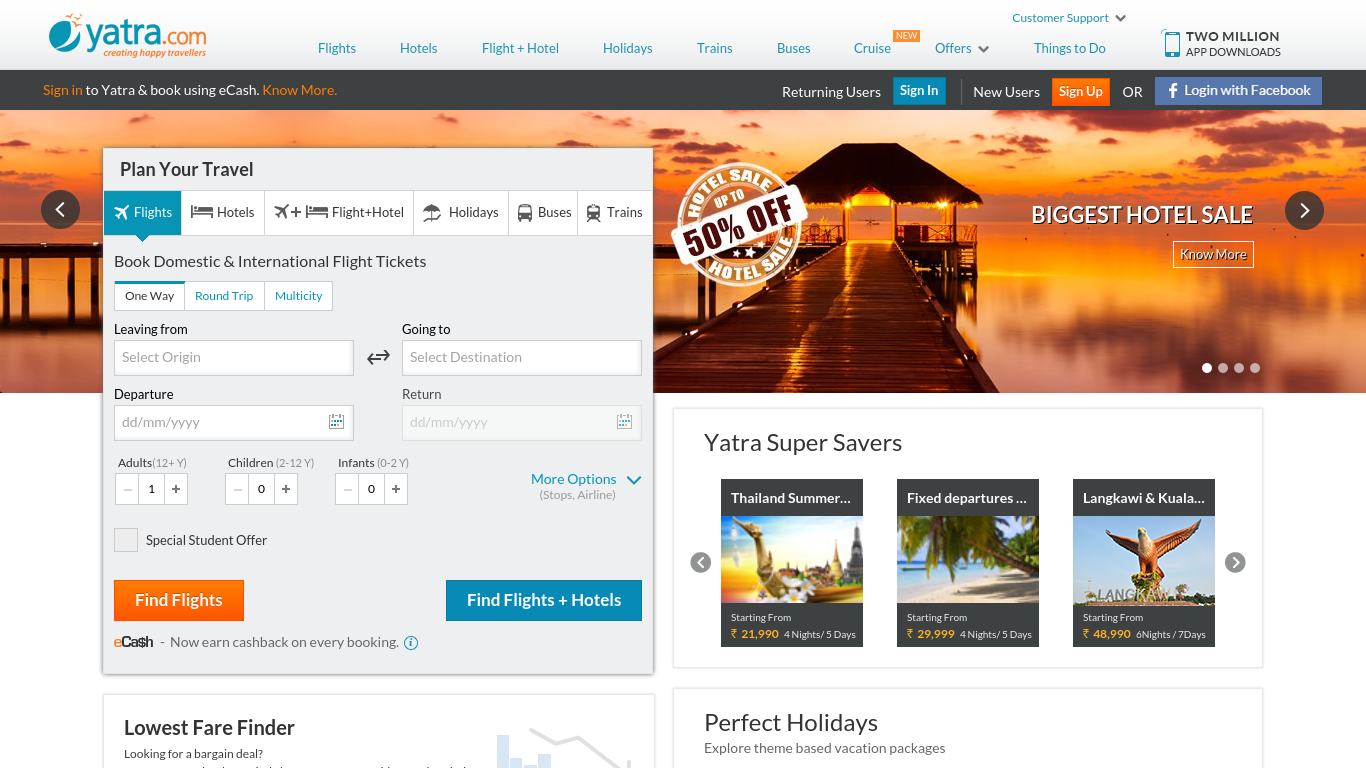A comprehensive view of a vacation booking website, Yatra.com, is displayed. In the upper left corner, the logo features a blue circle split in half with orange birds flying out of it, symbolizing the joy of travel. From left to right, the main headings offer various options including Flights, Hotels, Flight+Hotel, Holidays, Trains, Buses, and the newly added Cruise option. There's also an Offers section with a dropdown menu.

Below these headings, users can sign in or discover more about Yatra and book using eCash. On the right-hand side, returning users can quickly click the blue 'Sign In' button, while new users have the option to 'Sign Up' in orange or log in via Facebook.

Superimposed over an inviting sunset image with a boating dock and lights is a banner announcing a Hotel Sale of up to 50% off. On the left side, a 'Plan Your Travel' section features similar headings for Flights, Hotels, Flight+Hotel, Holidays, Buses, and Trains. The Flights option is activated, providing users with choices for One-Way, Round-Trip, or Multi-City travel. It offers fields to input the origin, departure, and return dates, as well as the destination airport.

In the center of this section, users can specify the number of Adult, Child, and Infant/Toddler travelers with convenient plus and minus buttons. Below these fields, prominent orange and blue buttons allow users to 'Find Flights' or 'Find Flights and Hotels,' streamlining the booking process.